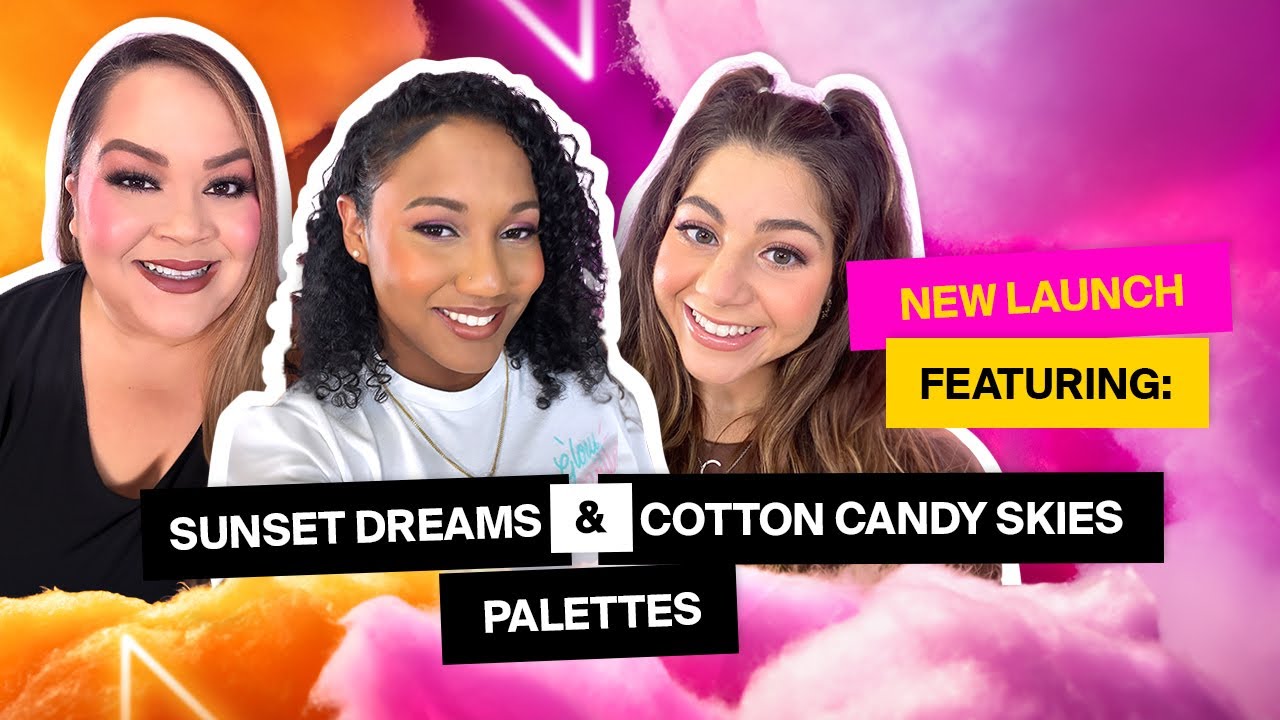This vibrant promotional image is an advertisement for a new makeup launch featuring the "Sunset Dreams" and "Cotton Candy Skies" palettes. The background transitions from left to right in hues of orange, purple, and pink, reminiscent of a dreamy cotton candy sky. The center of the image showcases three smiling women, each framed by a thick white border, exuding diversity and individuality.

On the left, a plus-sized woman with dark brown hair styled straight wears a black top. Her makeup is the darkest, emphasizing her features with bold eyebrows, intense eye makeup, and dark lipstick. The middle woman, an African-American with soft curly shoulder-length hair, dons a white crew neck t-shirt and a necklace. Her makeup is subtle and natural, harmonizing beautifully with her complexion. The woman on the right, the youngest of the trio, has long brown hair pulled into two playful pigtails, enhancing her youthful appearance. She sports a white top, a generous smile, minimal makeup, and a hint of lip gloss.

Overlaying the image is a thick black rectangle with the bold text "Sunset Dreams and Cotton Candy Skies." Below it, in a clean font, the brand name "Palettes" is printed, accompanied by "New Launch" in pink and "Featuring" in yellow, emphasizing the excitement of this fresh collection.